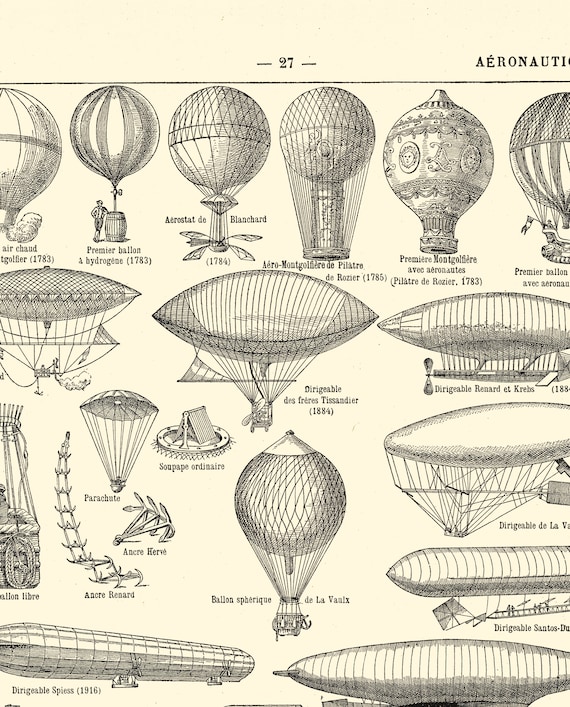This detailed and vintage pen-and-ink drawing is laid out on an ivory or old-fashioned yellowy beige background, characteristic of page 27 from an antique aeronautical book. The partially visible header spells out "AERONAUTICS" and features a numerical indication, "- 27 -". Spanning the entire page, the illustration showcases a variety of hot air balloons, blimps, and parachutes, meticulously labeled with their respective names and historical dates, such as the balloon from 1783. The images are organized into multiple rows: the top row displays six circular balloons, followed by a row of three almond-shaped balloons, and subsequent rows feature diverse designs including individual components like parachutes. A figure of a man standing next to one of the balloons adds a sense of scale. The detailed sketches reflect the evolution of aerial craft and offer a spectacular glimpse into the advancements in aeronautical design through different time periods.